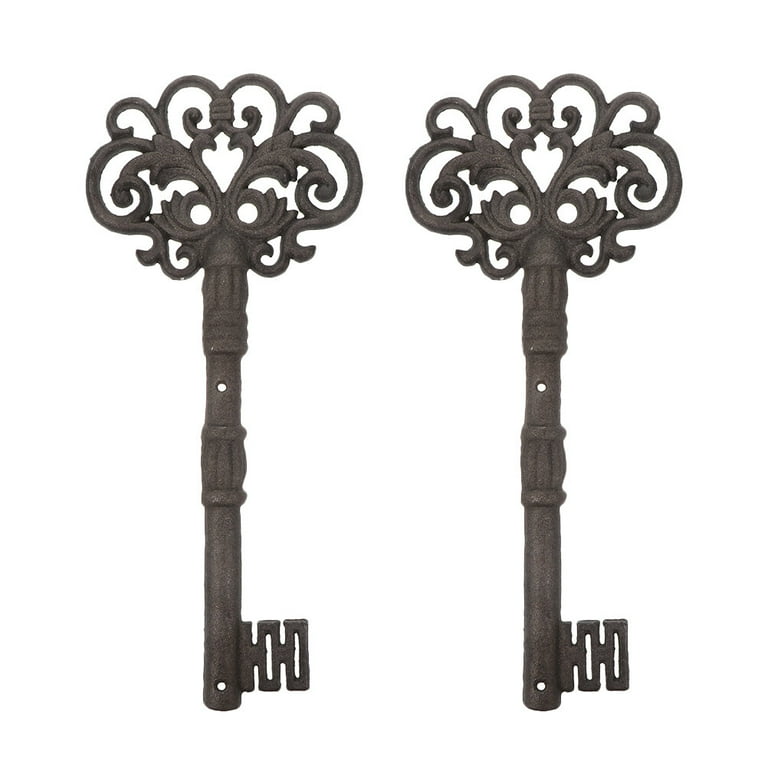The image features two identical vintage-style skeleton keys positioned vertically on a white background. Both keys are black, possibly cast iron, with intricate, decorative handles at the top. The handles boast detailed loops, swirls, and heart-shaped designs, giving them a frilly, calligraphic appearance reminiscent of old-time craftsmanship. The key's shaft extends downward to the actual bit, which consists of three rectangles: the first and third fully closed, while the second and fourth feature hollowed-out centers, giving the impression of interconnected squares. The keys lie parallel to each other, centered in the image, with no writing or additional elements, highlighting their elegant and ornate design against the stark white backdrop.